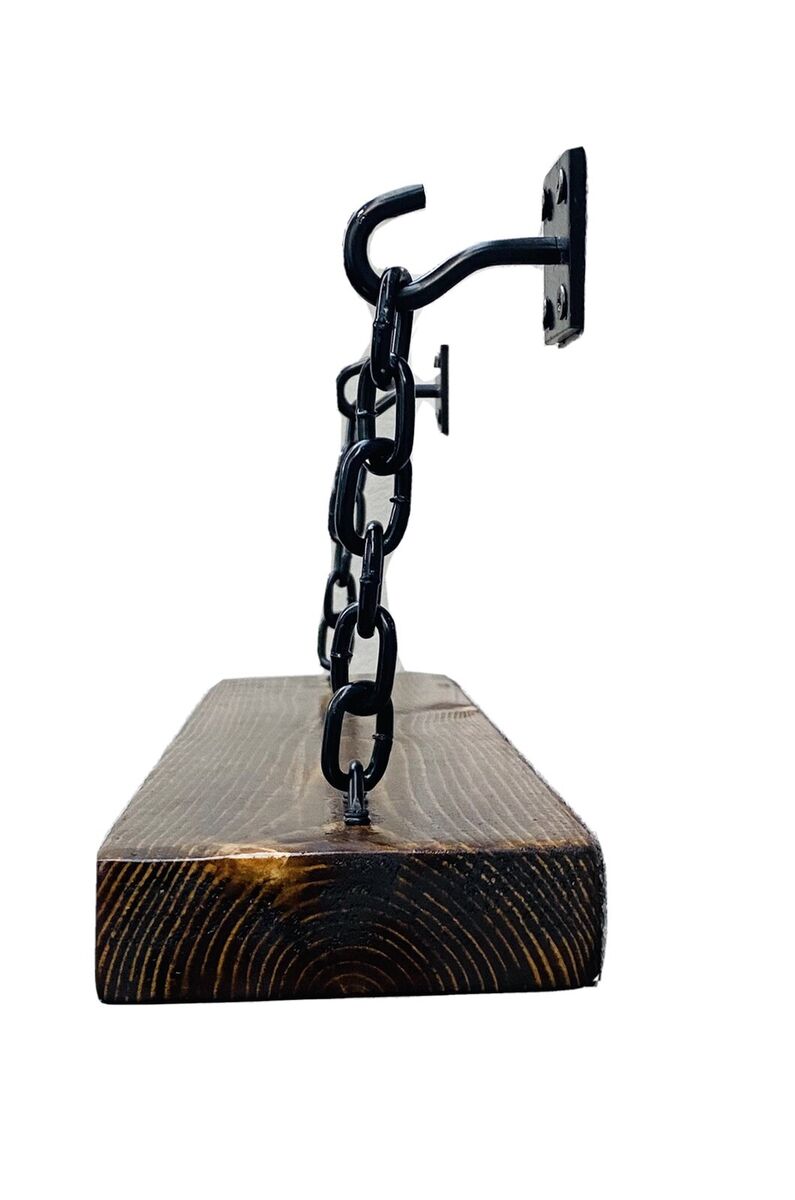This image features a side view photograph of a suspended shelf against a white background, showcasing its detailed construction and materials. The shelf is a long, rectangular piece of dark-stained wood, with visible tree rings emphasizing its natural grain. The darker stain has a deep, rich brown hue, with no hints of cherry or red, and exhibits slight wear in some areas where lighter wood peeks through.

The shelf is supported by short black chains, each consisting of five links that connect the shelf to black hooks mounted on the wall. These hooks extend straight out from the wall before curving upward to hold the chains securely. The hardware, including the black screws attaching the hooks, complements the overall dark aesthetic. The setup suggests that the shelf is leveled and firmly anchored, though it currently holds no objects.